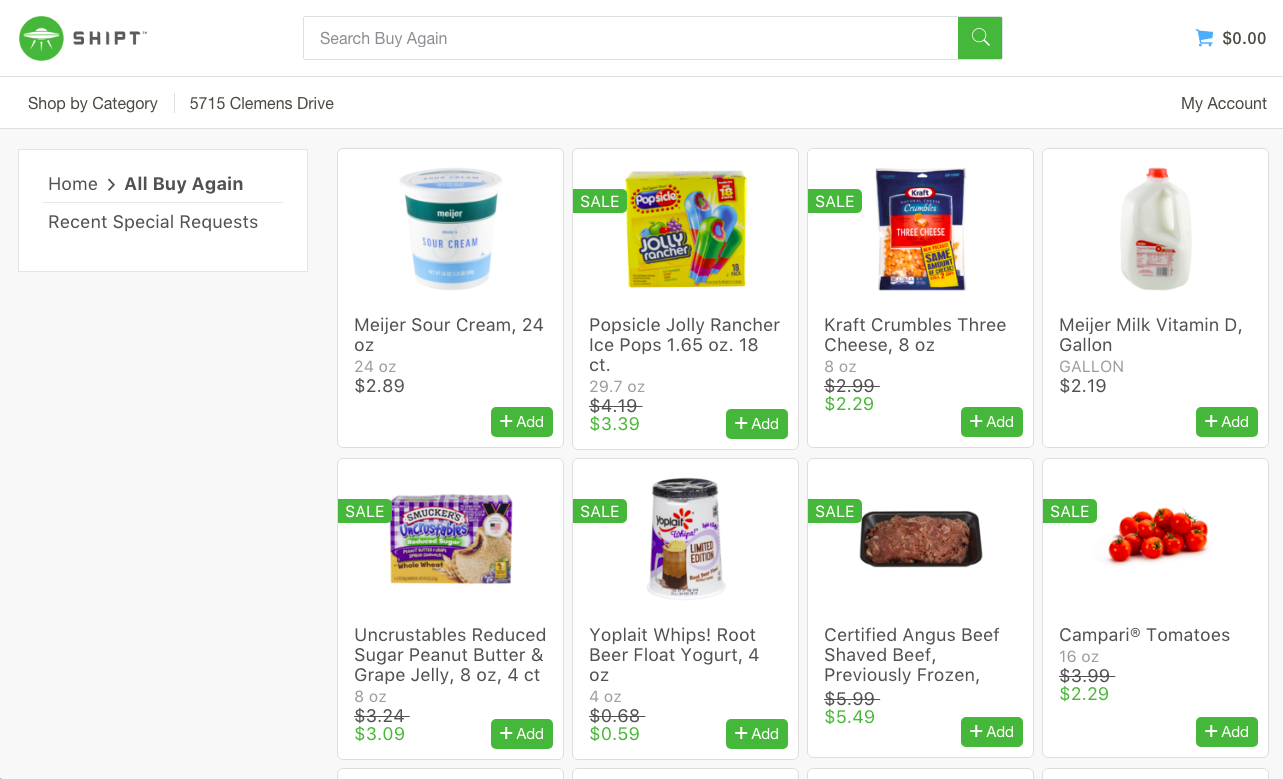Screenshot of a Shipt Grocery Ordering Page

The screenshot showcases a user-friendly interface from the Shipt grocery delivery service, featuring the brand's distinctive logo that includes the text "S-H-I-P-T" accompanied by a small alien spaceship decal. The page offers a wide selection of groceries, allowing you to purchase various items conveniently. Visible products include sour cream, popsicles, cheese, milk, tomatoes, and high-quality Angus beef. Additionally, it features Yoplait yogurt, reduced sugar peanut butter, and Smucker's grape jam. Each product is presented with a clearly marked green button, adorned with a plus sign, making it easy to add items to your shopping cart. The page also includes a search bar at the top for streamlined navigation, ensuring a hassle-free shopping experience. The overall layout is attractive and functional, designed to facilitate quick and efficient grocery selection and purchase.